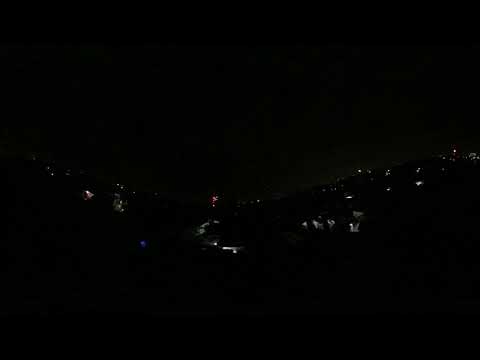The image is an almost completely black photo dominated by darkness, with minimal visible features. In the center, a silhouette of a hill descends from the left, dips in the middle, and ascends slightly to the right. This hill appears to be studded with tiny white lights, perhaps representing streetlights or apartment lights. The image gives off a sense of a distant landscape or neighborhood, possibly viewed through a fisheye lens, which may account for slight distortions. The lights are faint and scattered, making up the only discernible elements in an otherwise obscured and dark scene with no people, homes, words, or numbers visible.